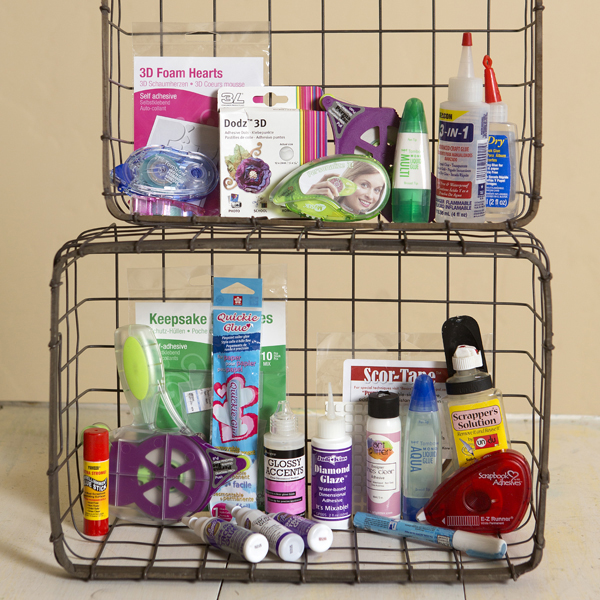This image depicts two wire baskets set on a concrete floor against a beige wall. The baskets, made of a lattice of thin wires, are positioned on their sides with a smaller one atop a larger one, partially cut off at the top of the frame. Both baskets are filled predominantly with craft supplies, though some items appear to be general office supplies.

In the upper, smaller basket, which includes a package of self-adhesive 3D foam hearts with a pink label on a white background, and a bottle of 3-in-1 spray adhesive among other miscellaneous items not easily identifiable.

The bottom, larger basket contains several types of glue, such as glossy accents glue, diamond glaze, water glue, and a glue stick. Additionally, there is scraper solution, quickie glue, and various types of tape, including a red plastic container of tape adhesive. There's also a pen and some other small, hard-to-identify objects.

Though the baskets and items might typically be found in a craft supply store or a small goods emporium, the precise labels on many products are difficult to discern, blending a mix of office and crafting materials displayed in a somewhat casual, cluttered arrangement.